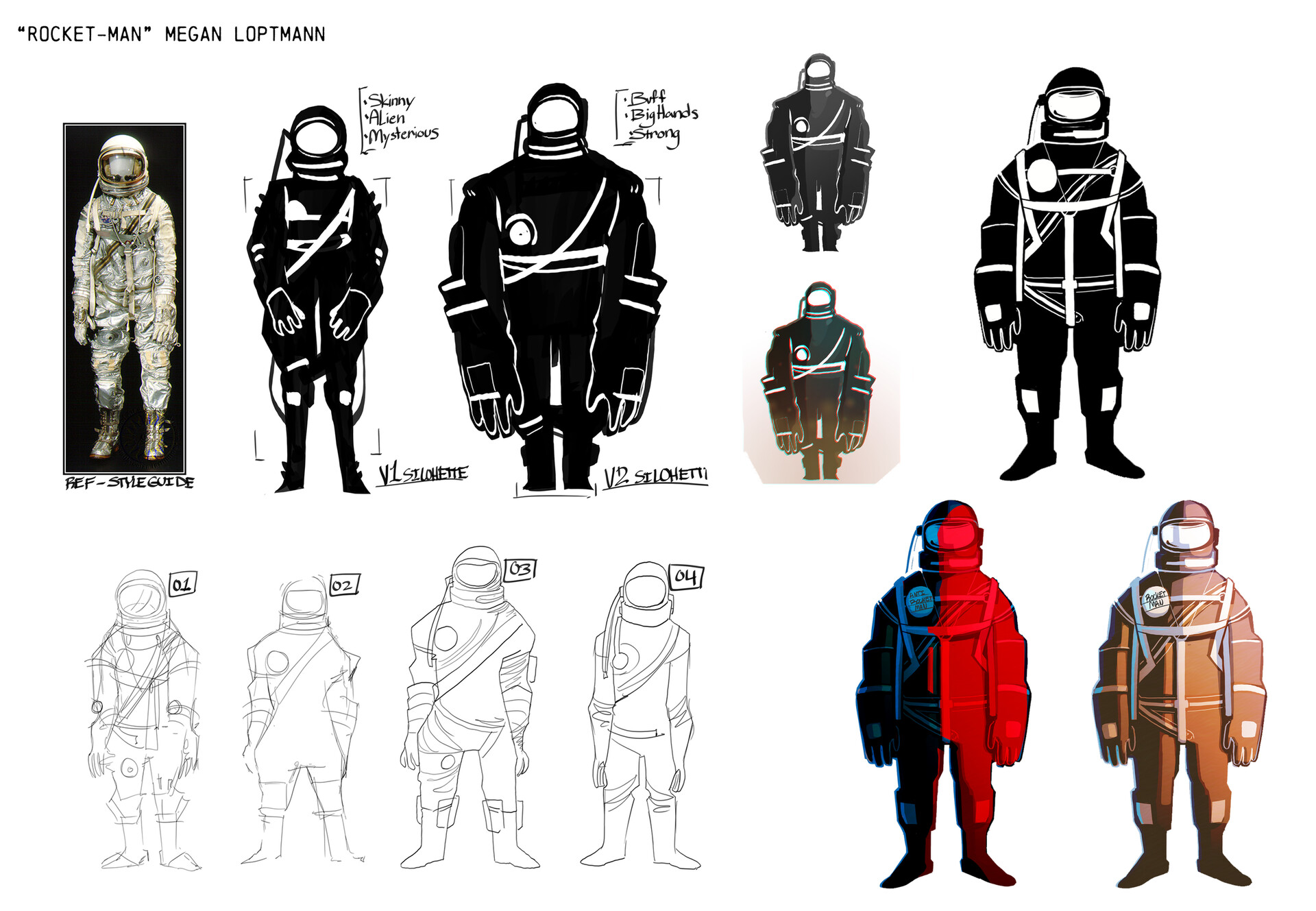The image showcases a series of detailed character model drawings titled "Rocketman Megan Loptman," with the artist's name prominently displayed at the top left. Below this title, the finished character model—a person in an astronaut suit adorned with numerous belts and thick, textured shoes—stands out. A small tassel extends from the right side of the helmet. The character's face is obscured by black helmets with white masks, adding a sense of mystery.

The top half of the landscape-oriented image features five distinct depictions of the spacesuit, all predominantly in black and white, except the first one, which is in color. These depictions include labeled silhouettes describing different body types (e.g., "V1 Silhouette, Skinny Alien Mysterious" and "V2 Silhouette, Buff, Big Hands Strong"). Additionally, one of the images in this row combines two smaller versions.

The bottom row presents four numbered outline sketches, followed by two colored illustrations: one with a suit painted blue on the left and red on the right, and the other with a brown suit. The design of the spacesuit is consistently depicted across all variations, with an emphasis on its intricate details and robust appearance.